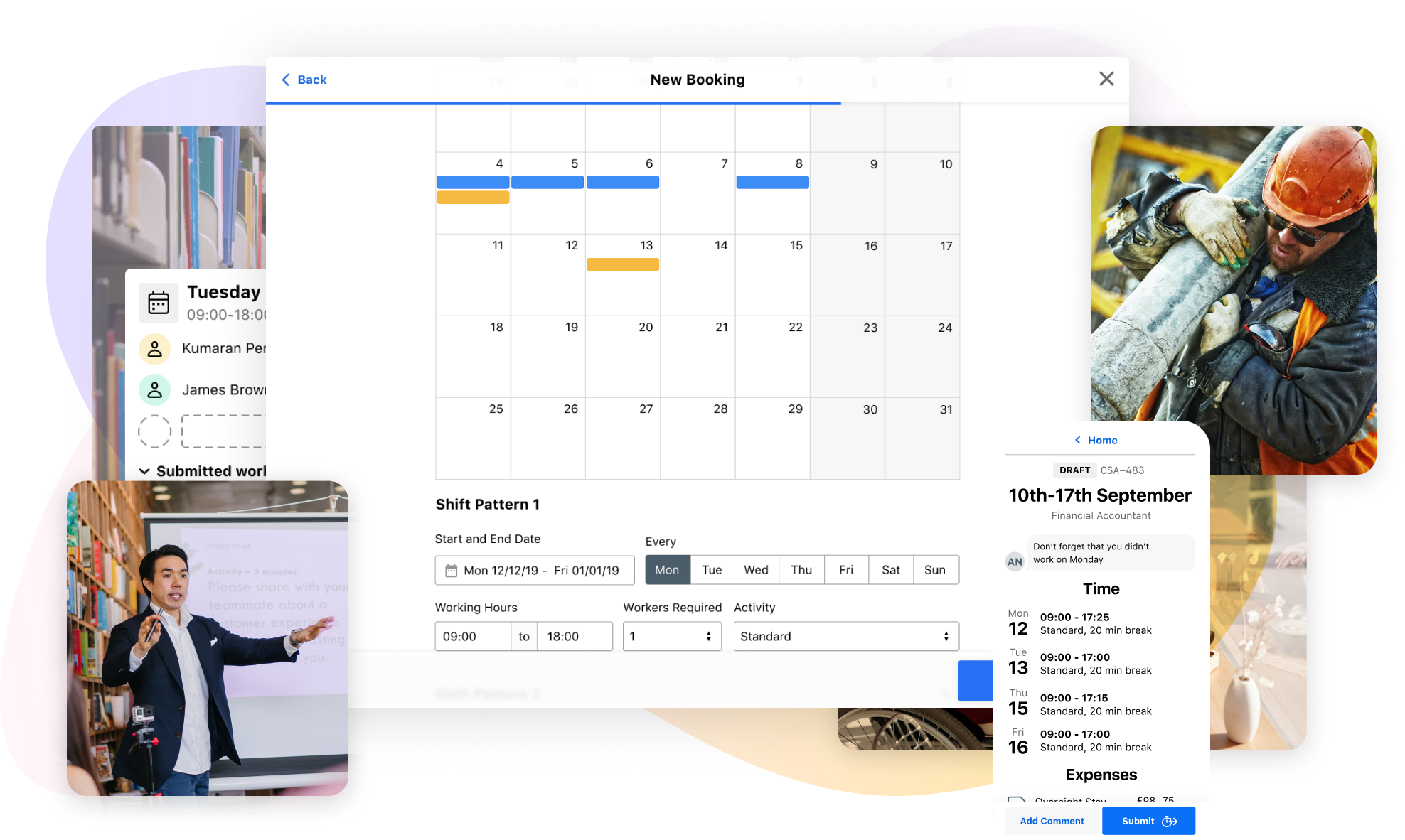The image features a central calendar labeled "New Booking" with navigational elements such as a back option in the top-left and a close (X) button in the top-right. The calendar begins on the 4th, which is the first day of the week, possibly a Sunday or Monday. Several dates, including the 4th, 5th, 6th, and 8th, are marked with blue rectangles, while the 4th and the 13th also feature goldish-yellow rectangles. 

Below this calendar is a section titled "Shift Pattern 1" that includes inputs for scheduling start and end dates, which are pre-filled with suggested dates from Monday, December 12, 2019, to Friday, January 1, 2019. Further options include selecting workdays, working hours, workers required, and activities. Beside this section is a smaller window showing a draft schedule from September 10th to 17th, detailing times for each day.

Overlapping the top-right corner of the calendar, there is an image of a construction worker outdoors, wearing an orange hard hat and sunglasses, and holding a heavy pipe. Behind and slightly beneath the calendar is an aesthetically pleasing shot of flowers in a vase.

In the bottom-left corner of the screen, a professor in a white shirt and a navy blue or black blazer stands mid-sentence, with his hands extended in front of him. He is positioned in front of a projector screen and bookshelf. Above this image and partially obscured by the professor and the calendar is another calendar-like item, displaying contact information and availability for "Tuesday 9 to 1800".